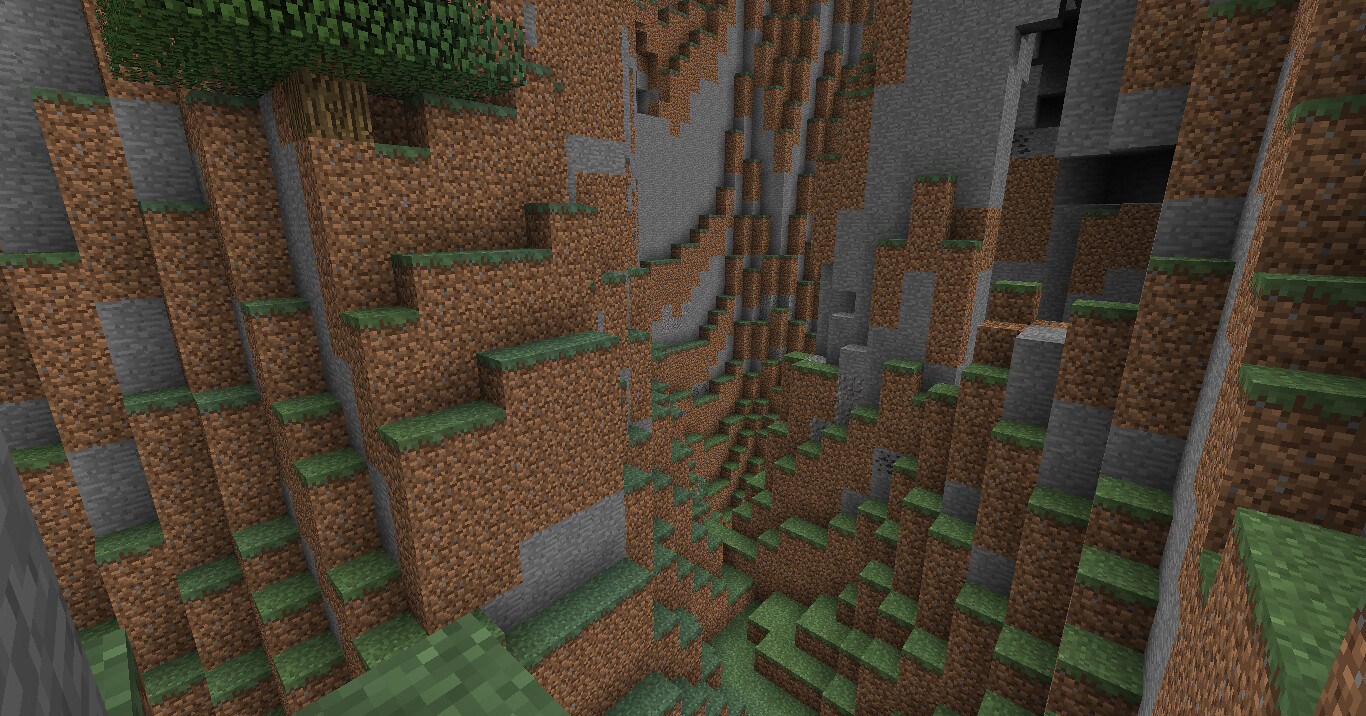This image is a screen capture from the popular video game Minecraft. It depicts a vast and expansive pit with towering cliffs and ledges that ascend dramatically. The ledges are primarily composed of brown and gray blocks, typical of the game's aesthetic, with patches of green grass crowning the upper surfaces of the brown blocks. The arrangement creates a sense of immense depth and complexity, with ledges scattered throughout the scene. In the background, the ledges seem to rise in a curved pattern, becoming denser towards a focal point, enhancing the impression of grandeur and scale.